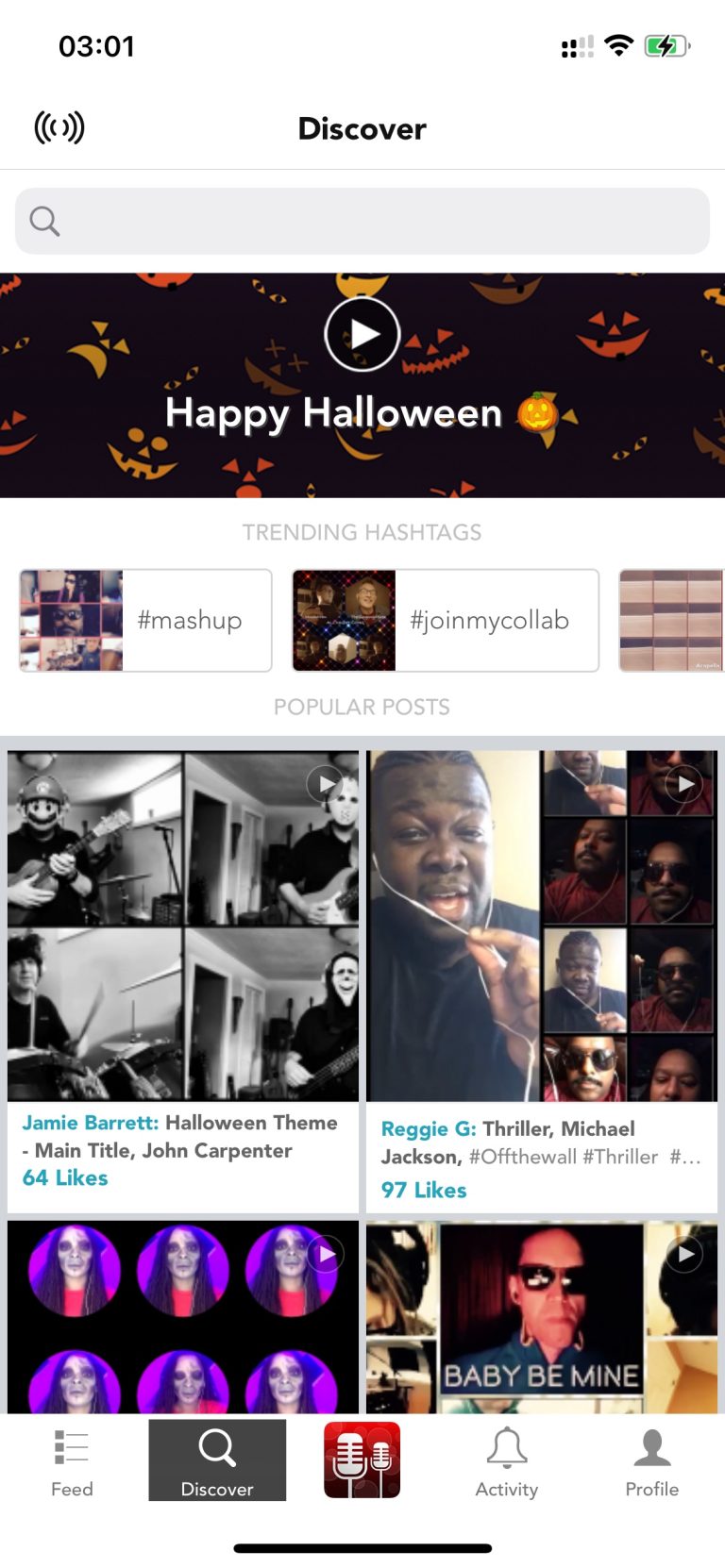In this image, the top part features the black text "Discover" against a white background. Directly beneath this heading, there is a search bar. Below the search bar lies a video thumbnail with a play button, and the words "Happy Halloween" are displayed prominently. Surrounding the play button are various smiley faces in orange and yellow, each displaying different expressions—some happy, some sad, some with perfect teeth, others missing teeth. Also, a yellow pumpkin with a carved smiley face is present.

Underneath the video section, the text "Trending Hashtags" appears, highlighting two hashtags: #mashup and #joinmycollab. Following this, the "Popular Post" section showcases four posts. The top two posts include descriptions, while the bottom two have hidden descriptions.

The top left post is by Jamie Barrett with a Halloween theme, titled "Main Title," attributed to John Carpenter, and has garnered 64 likes. Both the name and likes are in blue, with the description in black. The top right post, by Reggie G, is centered around Michael Jackson's "Thriller" and includes hashtags #offthewall and #thriller, with 97 likes indicated in blue.

At the very bottom of the image, there's a row of buttons. On the bottom left are "Fit" and "Discover," with "Discover" highlighted in grey and "Fit" drawn in grey. The center features a white microphone icon against a red background. On the bottom right are the "Activity" and "Profile" buttons, both in white.